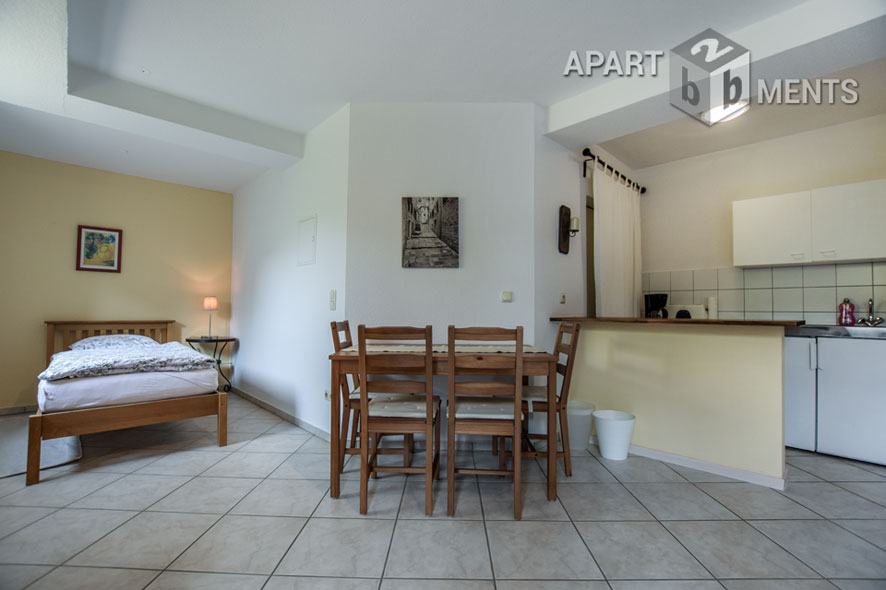This is an image of a compact studio apartment featuring a seamless layout without walls dividing the space. To the left, there is a small bedroom area with a brown wooden bed frame, complete with a headboard and footboard, dressed in a white sheet and a grayish-white comforter. A nightstand with a lamp sits nearby, and a picture frame with blue and yellow hues is centered above the bed against a yellow-painted wall.

Adjacent to the bedroom, in the middle area, there is a small dining setup with a square table and four wooden chairs that have beige seat covers. A picture hangs above this dining area, adding a touch of decor.

To the right, the apartment transitions into a compact kitchen area. The kitchen features white cabinets both above and below the sink, white tile backsplash, and countertops likely made of aluminum or stainless steel. A white bucket is noticeable near the sink area, and a pantry is concealed with a curtain that can be opened and closed by hand. Additionally, there is a plaque or sconce with a candle to the left of the pantry curtain. The overall scheme of the apartment is accentuated by beige-colored square tiles on the floor, and the ceiling and walls are painted white, adding to the brightness of the space. In the upper right-hand corner, there is a unique decoration with the word "apartments" split by a cubicle shape containing the letters 'B' on either side and the number '2' on top.